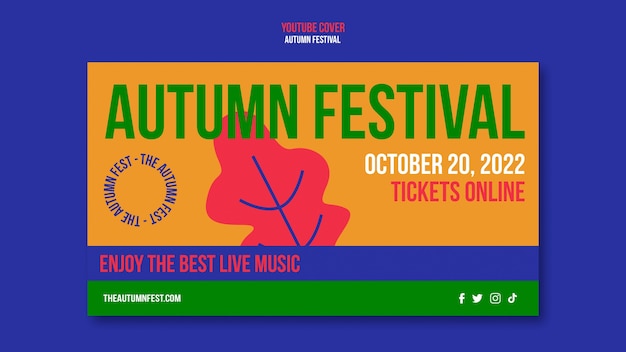This image is a detailed advertisement for an Autumn Festival. The background is composed of a large purple rectangle. At the top center, there is text in red font that says "YouTube Cover." Directly below this, in white font, it reads "Autumn Festival."

Beneath the initial purple rectangle is an orange rectangle. At its top, in red font, the words "Autumn Festival" are displayed again. Below this, there is a graphic of a dead leaf, which is brown with a blue vein running through it. 

To the left of the leaf, there is a circular design with blue text that repeatedly says "The Autumn Fest" in a circular pattern. To the right of the leaf, in white font, it states "October 20th, 2022." Below this date, in green font, it says "Tickets Online."

Continuing downward, another purple rectangle appears with red font inside it, which reads "Enjoy the Best Live Music." Immediately below this text is a green rectangle with white font, displaying "The Autumn Fest."

On the right end of the advertisement, there are four white social media icons for Facebook, Twitter, Instagram, and TikTok.